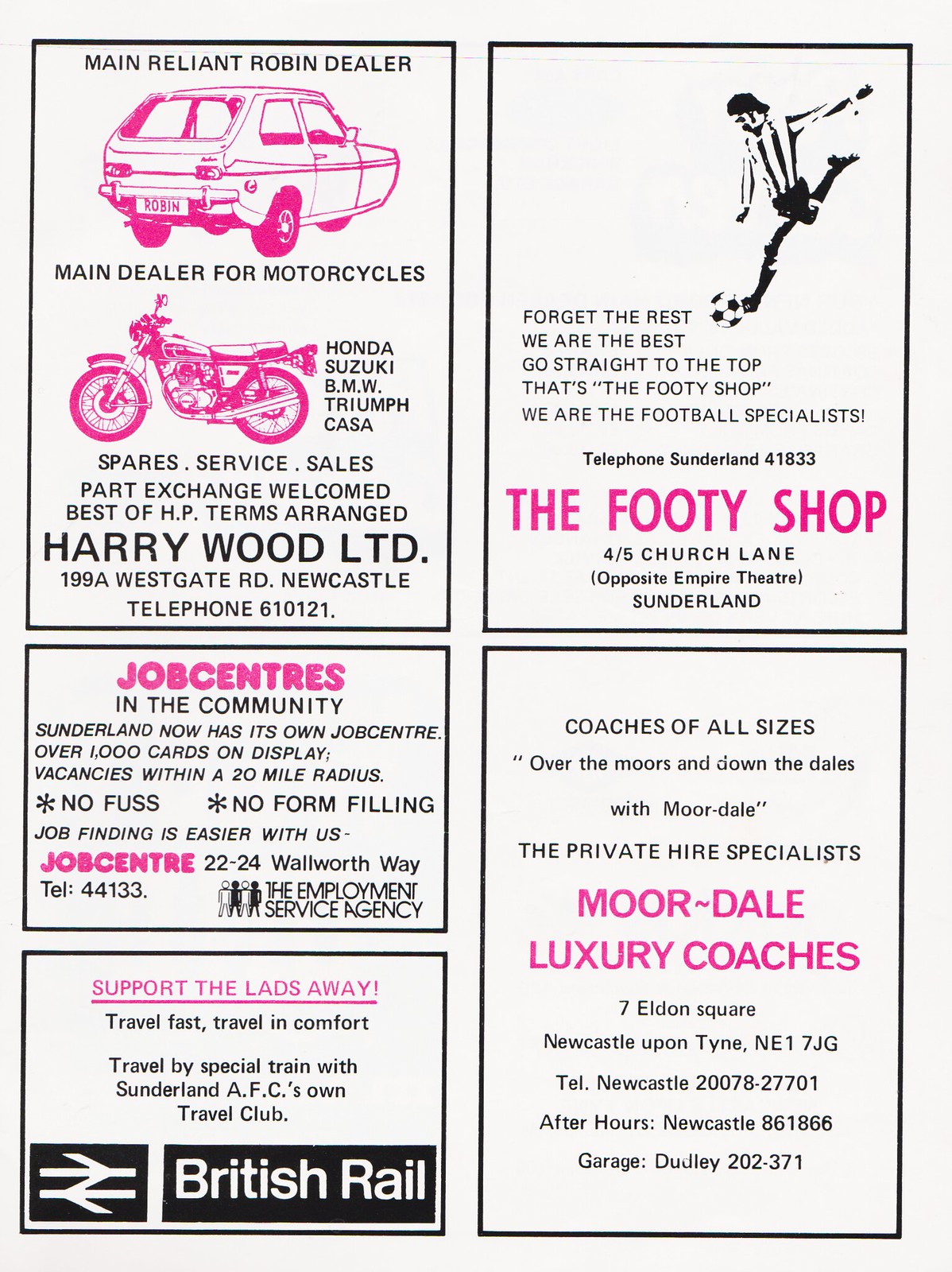This page from a soccer magazine features a collection of advertisements in black and magenta on a white background, all enclosed by black borders. At the top left, the main ad for Harrywood Ltd. highlights their status as the Main Reliant Robin Dealer and Main Dealer for Honda, Suzuki, BMW, Triumph, and Kasa motorcycles. It includes an eye-catching magenta illustration of a Reliant Robin car and a motorcycle. The text mentions their services: spares, service, sales, and car exchange, with a welcoming note on HP terms arranged. Their address is 199A Westgate Road, Newcastle, and their telephone number is 610121.

Beneath this, an ad for the local job center states Sunderland now boasts its own job center with over 1,000 job cards on display, covering vacancies within a 20-mile radius, promising ease in job finding with no fuss or form filling. Located at 22-24 Walworth Way, Sunderland, their telephone number is 44133.

To the right, the top ad promotes ‘The Footie Shop’ with an image of a man poised to kick a soccer ball. The catchy slogans, "Forget the rest, we are the best" and "Go straight to the top, that’s the Footie Shop," emphasize their expertise in football, located at 4-5 Church Lane, opposite Empire Theatre, Sunderland, with a contact number of 41833.

Directly below, a supportive ad encourages fans to "Support the lads away" by traveling fast and comfortably with Sunderland AFC’s own Travel Club via British Rail.

In the bottom right corner, Moordale Luxury Coaches advertises their private hire services with coaches of all sizes. The ad reads, "Over the Moors and Down the Dales with Moordale," reinforcing their speciality and providing their address at 7 Eldon Square, Newcastle upon Tyne, NE1 7JG, with telephone numbers 20078-27701 and after-hours contact 861866.